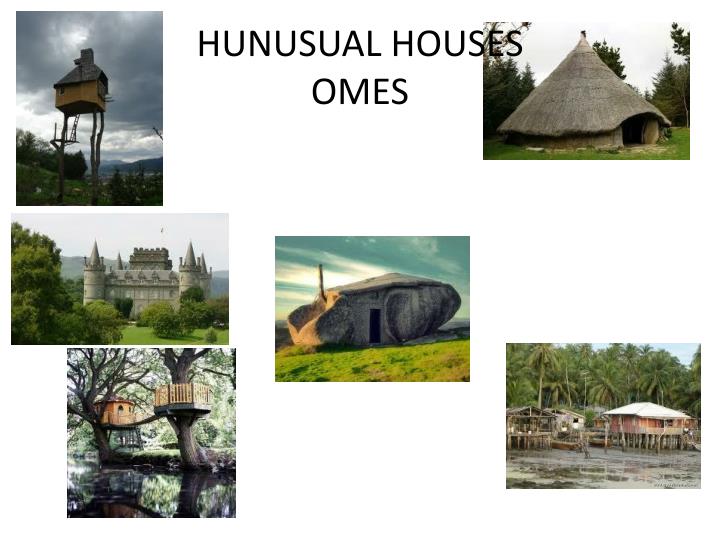The image features a white background with six photographs arranged within an implied rectangle, where the left and right sides are shorter than the top and bottom. In the center top, the text "Unusual Houses Owns" appears in indistinct uppercase black letters. Each photograph captures an extraordinary type of house.

1. **Top Left:** A perfect square photograph of a small hut or house on very high stilts. The structure appears to have tan walls, a gray thatched roof, possibly a chimney, and is set against a gradient gray sky with black silhouettes of trees or buildings in the background.

2. **Middle Left:** A horizontally aligned rectangle showcasing a white castle with red roofs, pointed towers at each corner, numerous balconies, and a grid of windows. The castle is surrounded by lush greenery with hills and a light blue sky featuring a distinct grove of trees.

3. **Bottom Left:** A double-structure treehouse over a reflective river or lake. The left side features the main treehouse with rounded walls and a flat roof, connected by a bridge to a tree with a balcony on the right. The setting includes a small cliff-like bank and expansive foliage with a pale sky.

4. **Center:** A photo of a ship-like structure lying on its side on green grass, under a cold gray and white sky. The ship appears tan and brown, suggesting sunlight coming from the left, casting a shadow on the right side.

5. **Top Right:** A conical grass hut with a large entryway, mostly obscured by its extensive roof. It sits within a wooded area with a partially cloudy whitish-blue sky backdrop. The hut’s roof is textured and grayish, with very short walls, emphasizing its natural material composition.

6. **Bottom Right:** A beachside scene with a house on stilts partially submerged in water. This house is pink with a white roof. To the left, there appears to be wreckage or fallen trees, and the river beneath is swiftly moving. The background shows a blue sky and another structure that looks worn down.

These photographs collectively present a diverse array of unusual homes, each with distinct architectural and environmental features.